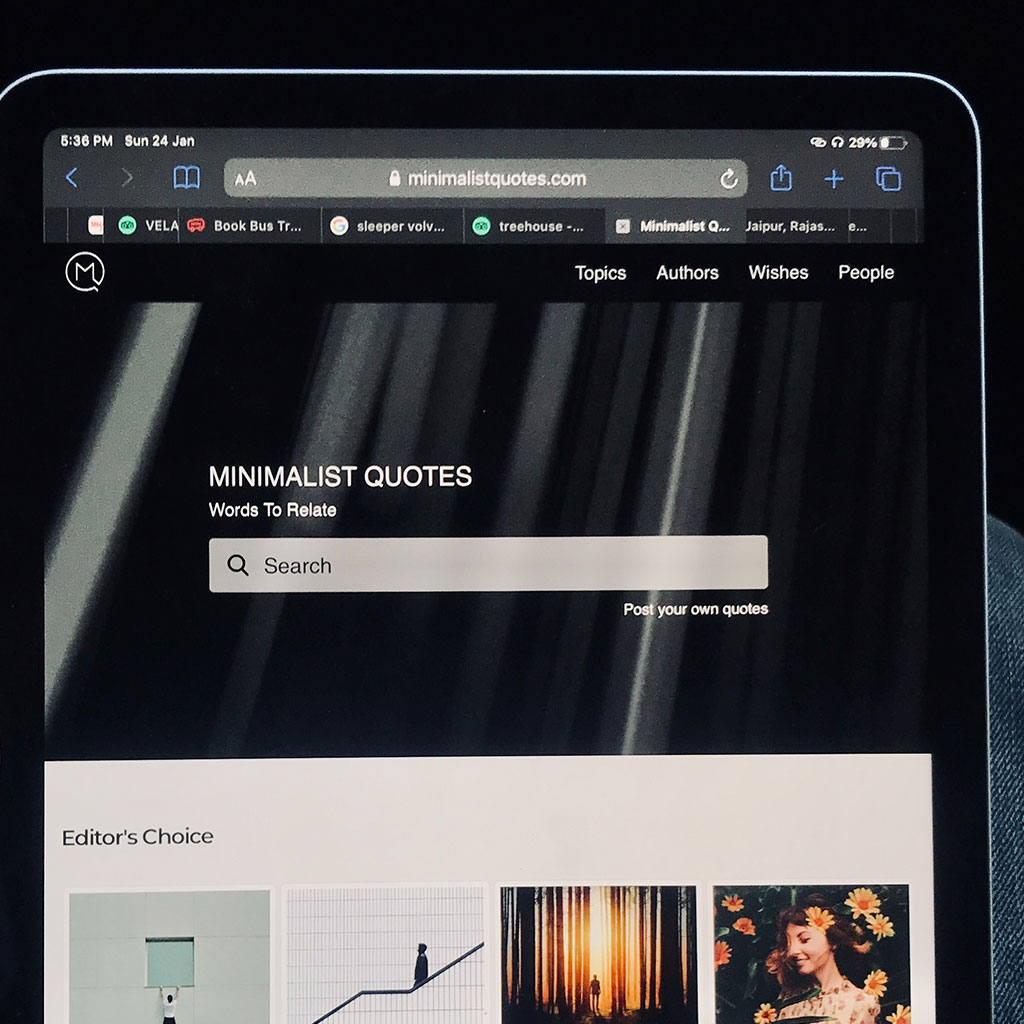A smartphone is positioned on the knee of an individual who is wearing denim, as indicated by the visible fabric in the bottom right corner of the image. The phone's screen prominently displays a grey notification bar at the top. On the left side of this bar, the current time shows 5:36 PM, and the date reads Sunday, January 24th. Centrally located in this grey panel is the website minimalistquotes.com, while the right side of the panel shows a battery icon with 29% remaining.

Below the grey panel, various tabs are visible, including "Villa," "Book Bus Trip," "Sleepers," "Treehouse," and "Minimalist Quotes," with the latter being the currently selected tab. On the right side beneath this panel is a black sidebar featuring headings: "Topics," "Authors," "Wishes," and "People."

Dominating the center of the screen is a search dialog set against a black, diagonally-striped background, inviting users to search for minimalist quotes. Beneath this, a link labeled "Post Your Own Quotes" offers user interaction. At the bottom of the screen, there are sections for "Editor's Choices" accompanied by corresponding images just above them.